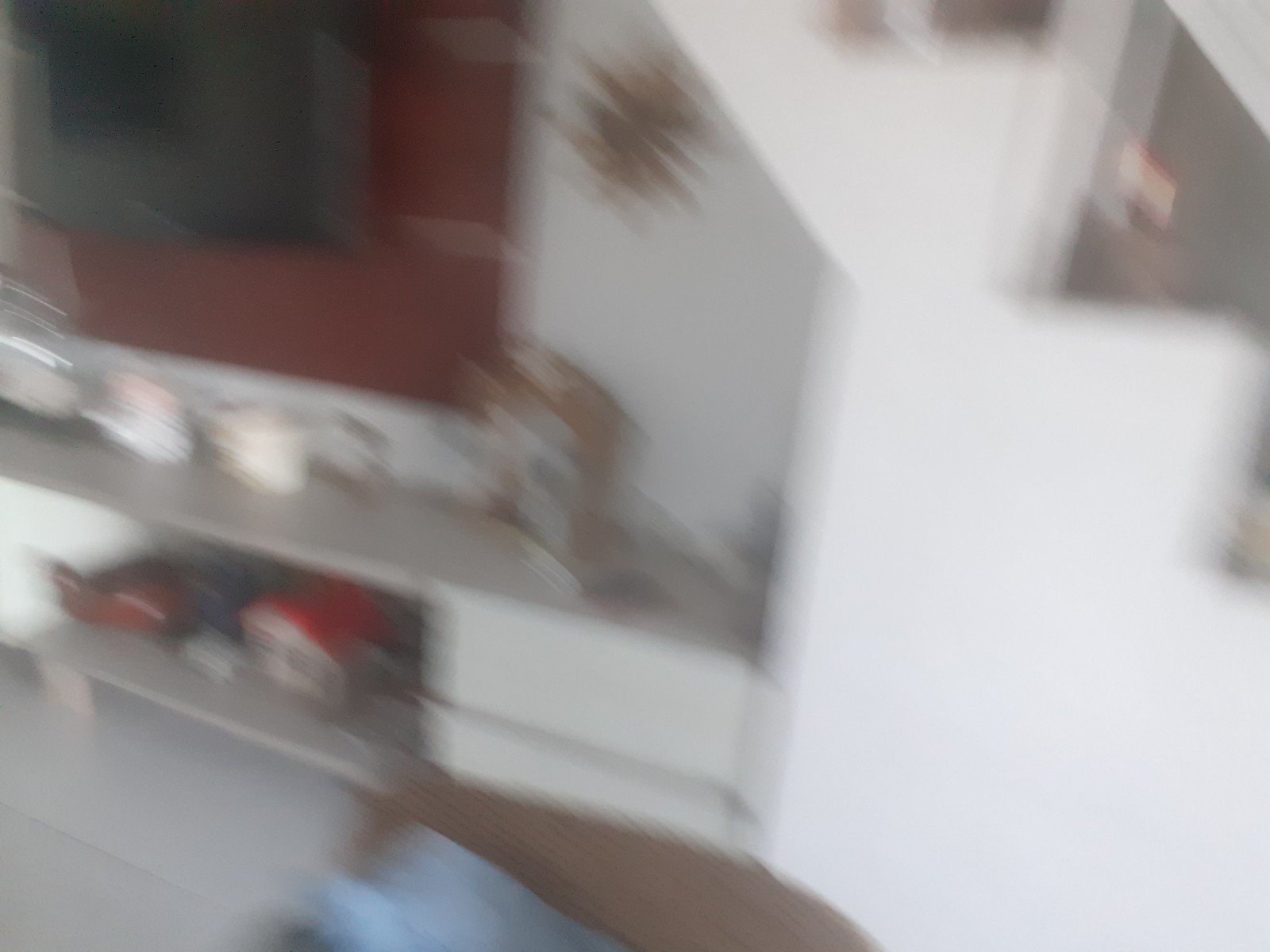The photograph, though blurry, appears to capture the interior of a living room. In the upper left corner, a wall-mounted television is visible, perched above a low, two-shelved cabinet designed to house electronic devices like a VCR. To the right, there is a stairway leading upwards, with pristine white walls providing a bright contrast. The back of the television has a brown hue, further setting it apart from the white wall. The flooring is adorned with white tiles, contributing to the room's clean and crisp appearance.